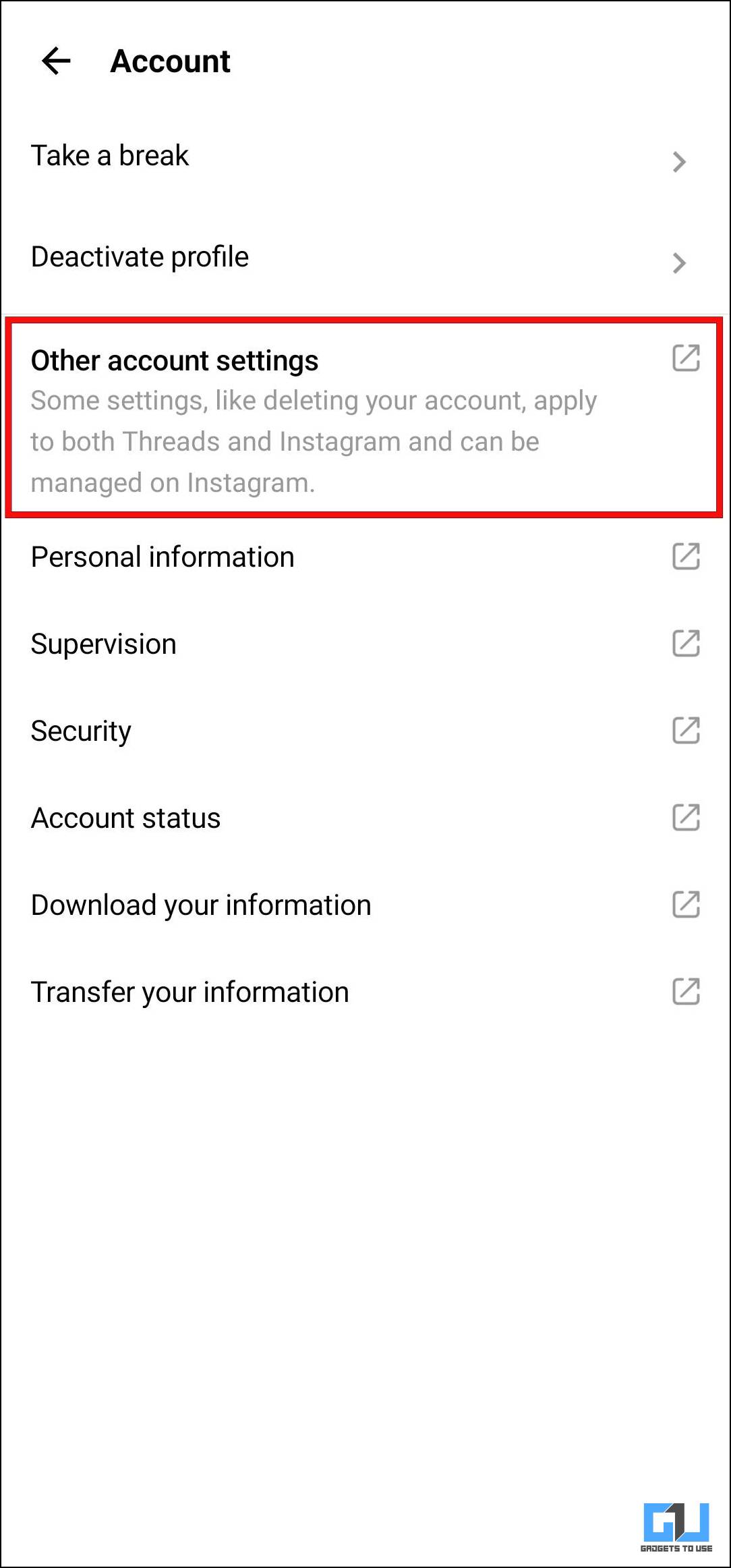The image displays a user's account settings page with a clean, white background. At the top-left corner is a leftward-pointing arrow, indicating a back navigation option. Bold black lettering reads "Account" as a header. 

Below the header, there is a listing of options starting with "Take a break," highlighted by a rightward-pointing arrow. Following that is "Deactivate profile," similarly denoted with a rightward-pointing arrow. 

One notable section is highlighted in a red box: "Other account settings." A description beneath it reads, "Some settings, like deleting your account, apply to both Threads and Instagram and can be managed on Instagram."

The page continues with a comprehensive list of additional settings, each item accompanied by a clickable area to the right for further navigation:
- Personal Information
- Supervision
- Security
- Account Status
- Download Your Information
- Transfer Your Information

At the very bottom of the page, there is a small logo followed by the letters "GU."